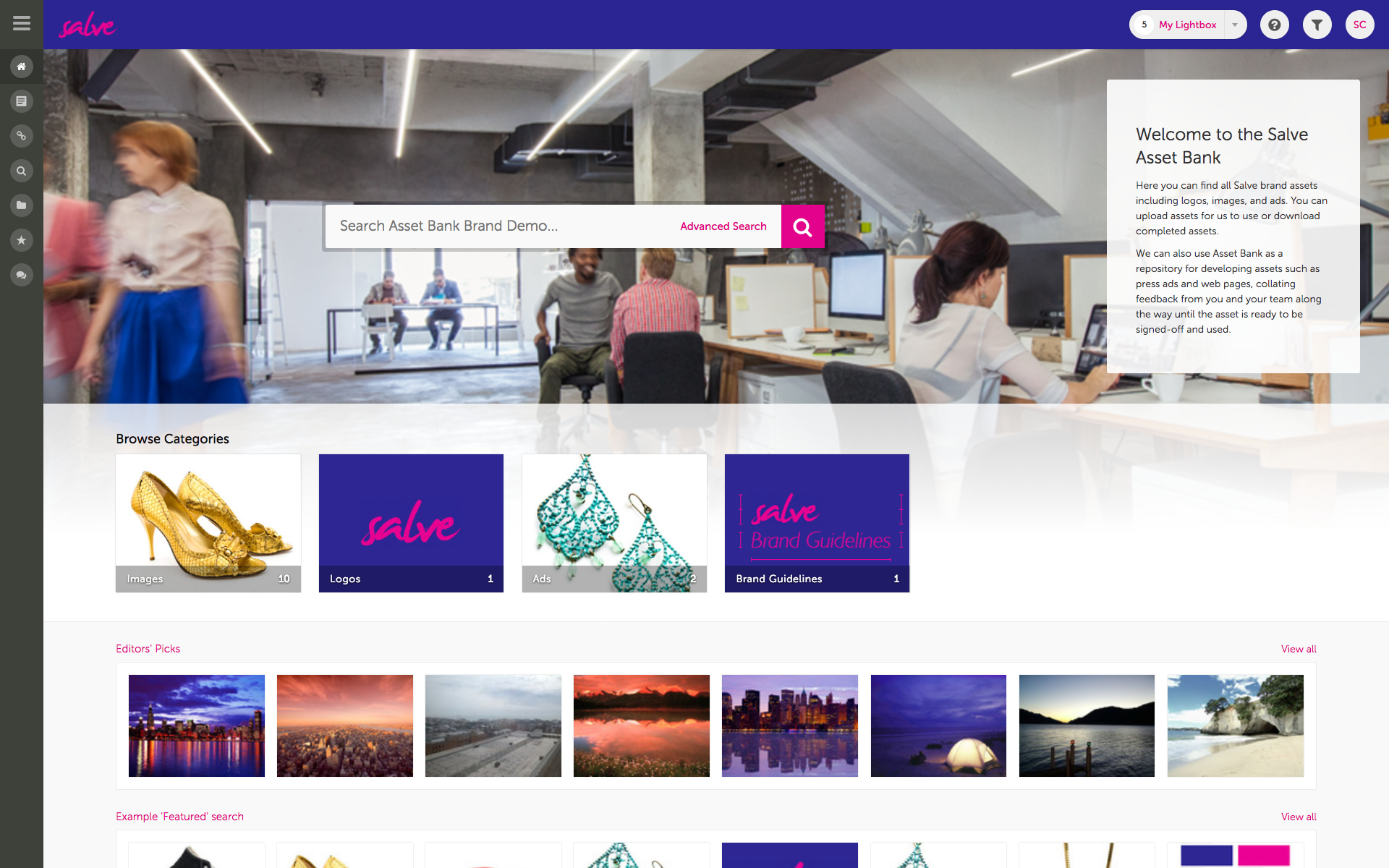The captured image features a partial view of the FASAV website, prominently displayed in a vibrant fuchsia color. At the top of the page, there's a navy blue stripe. On the left side, a black column with various options is visible, though it does not seem to be an integral part of the website. 

The upper section of the page showcases a photograph of a small office setting. In this image, two men and two women are seen, along with two other gentlemen seated at a long table in an adjacent open room. Below this, the 'Browse Categories' section is visible, displaying options like shoes, logos, ads, and brand guidelines.

Further down, the 'Editor's Picks' section features several images of diverse landscapes. Beneath this section, there's a glimpse of the 'Example Featured Search' area, though only the top edge is visible. To the right within the picture, the text "Welcome to the SAV Asset Bank" is displayed, accompanied by some additional text and a search bar strewn across the image.